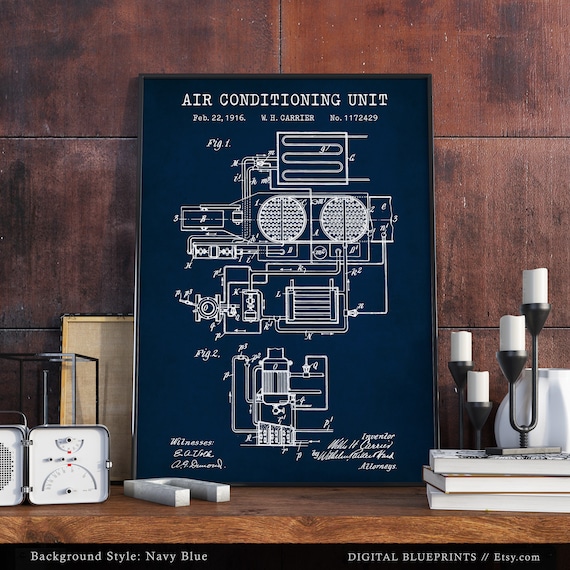The image depicts a detailed, photorealistic picture of a historical air-conditioning unit blueprint, dated February 22, 1946, attributed to W.H. Carrier, with the serial number No. 1172429. This intricately outlined blueprint is encased in an apparent black or brown frame and is centrally placed on a brown table against a dark brown, possibly tiled wall. 

The blueprint itself is set against a blue backdrop with white stenciling, which annotates various parts of the air-conditioning unit through numbered distinctions. Surrounding the framed image are diverse objects: to the left, a series of clocks or measuring devices, including a gauge-like machinery with a partial circle and arm. In the foreground, a white horseshoe-shaped tool is present. To the right, there are three books stacked upon each other, topped with four white candlesticks and accompanied by a small white jar.

Additional text at the bottom of the image reads: "Background Style, Navy Blue, Digital Blueprints, Hashtag Etsy.com." The meticulous representation of the mechanical parts captured in this diagram highlights the intricate inner workings of the air-conditioning unit.